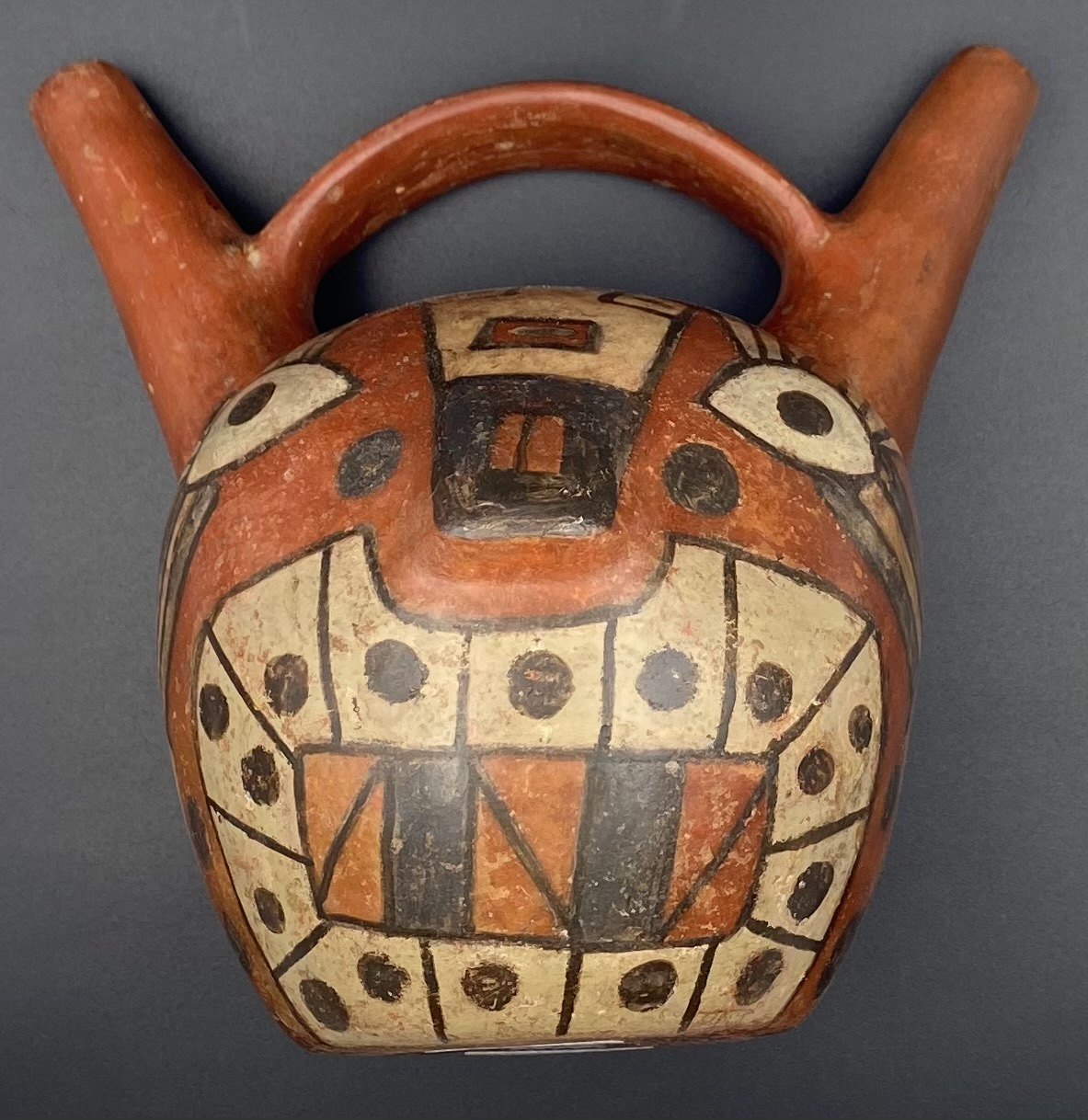This image showcases a handcrafted wooden artifact, likely representing a facial figure, with possible African or Egyptian influences. The base of the object is round and flat on the bottom, while the top features two protrusions resembling ears, which are connected by a curved handle. The face is artfully detailed, with white eyes outlined in black and centered with black pupils, giving it an expressive look. The nose is depicted as a black square with two vertical brown lines. The mouth area is surrounded by white squares with either one or two black dots inside, mimicking teeth. The overall color palette includes dark brown wood tones accented with whites, blacks, oranges, and grays. Some of the rectangular areas around the mouth incorporate diagonal lines and other patterns, suggesting a mix of traditional and modern artistic techniques, possibly using acrylic paint.